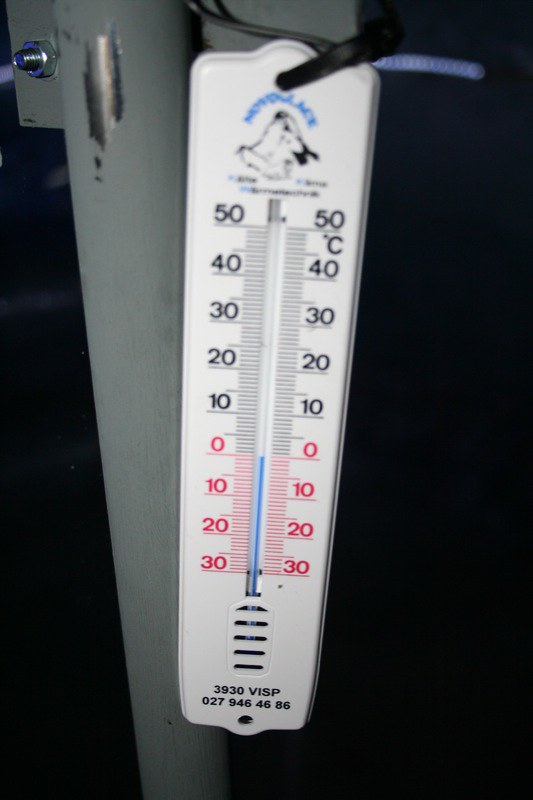This is a portrait-oriented photograph of a white thermometer, calibrated in Celsius, and mounted on an outdoor pole or post. The measurable range of the thermometer spans from -30°C to 50°C. The thermometer features slightly blurry brand or product markings at its top, making them illegible. The temperature scale displays red digits for readings below 0°C, transitioning to black digits for temperatures from 0°C and above. The scale includes numbers in 10-degree increments and has clear lines marking each degree, with more prominent markings for every half-degree, facilitating precise temperature readings. The image was captured at night, as indicated by the pitch-black background.